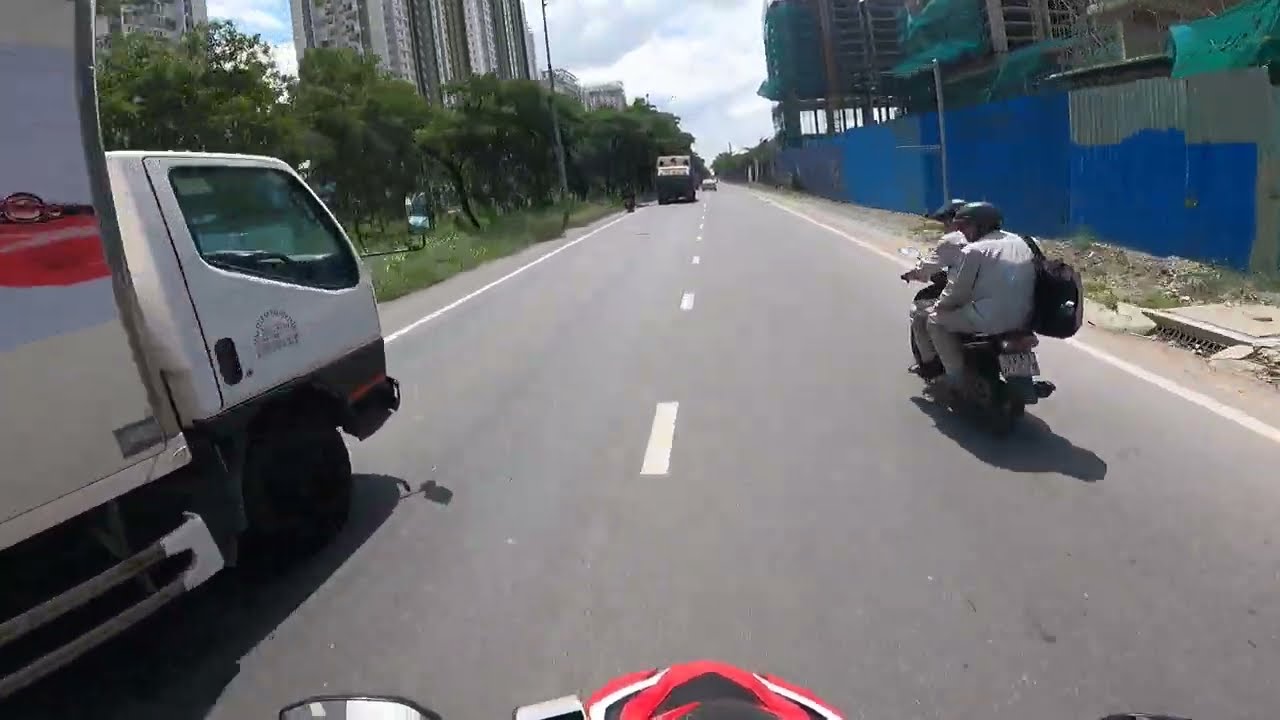This horizontal rectangular image, likely captured from a GoPro, shows a dynamic street scene featuring two people riding a scooter-type motorcycle on a two-lane road marked with white dashed lines down the center. Both riders are wearing helmets; the one on the back is dressed in a light-colored, long-sleeve shirt and tan pants, carrying a black backpack over their right shoulder. The road appears to be one-way, as cars and trucks in both lanes are traveling in the same direction. 

To the left of the motorcycle, there’s a white truck resembling a U-Haul with a partially visible red graphic. Further in the background on the left lane, there is another truck, and a motorcycle is parked on the shoulder. A car is visible in the distance further up the road. The right side of the road features a weathered fence with a mix of blue and gray paint, alongside some dilapidated buildings. Large, tall buildings and green trees can be seen lining the left side of the road. At the very bottom of the picture, part of another motorcycle is visible, showing a glimpse of its red front and the top of a left-side mirror.